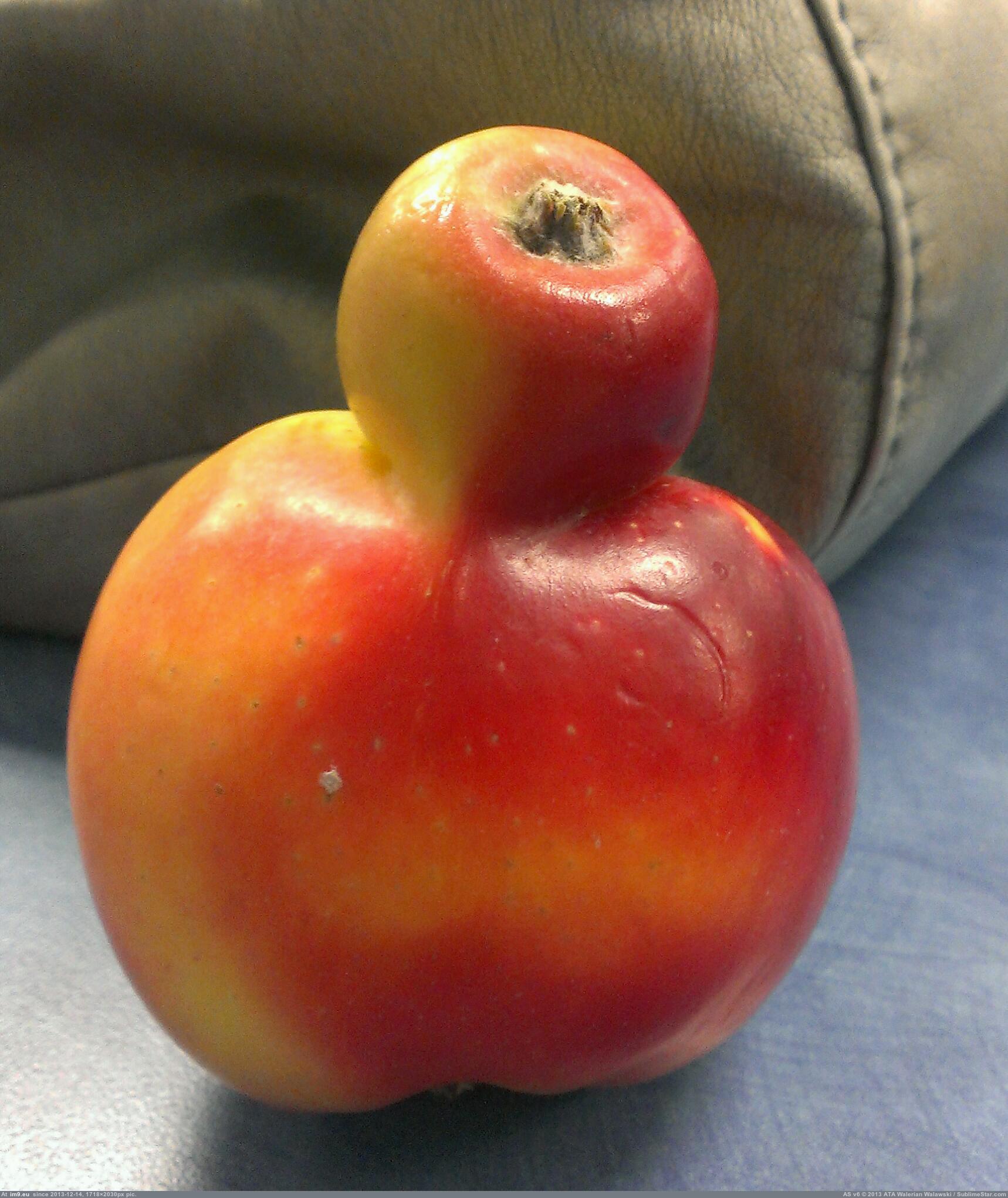This photograph, captured in portrait orientation, features an unusual-looking fruit placed on a blue surface. The main subject is a misshapen tomato, though it resembles an apple due to its unique form. The tomato is predominantly red and yellow with small brown or beige specks scattered across its surface. Noteworthy is the peculiar growth on top, resembling a smaller version of the fruit, as if a tiny tomato is sprouting from the larger one. The background showcases a brown, cracked leather bag, adding a texture contrast to the image. The bag has visible black stitching and cracks. At the very bottom of the image, a gray line runs horizontally, along with some unreadable white text.